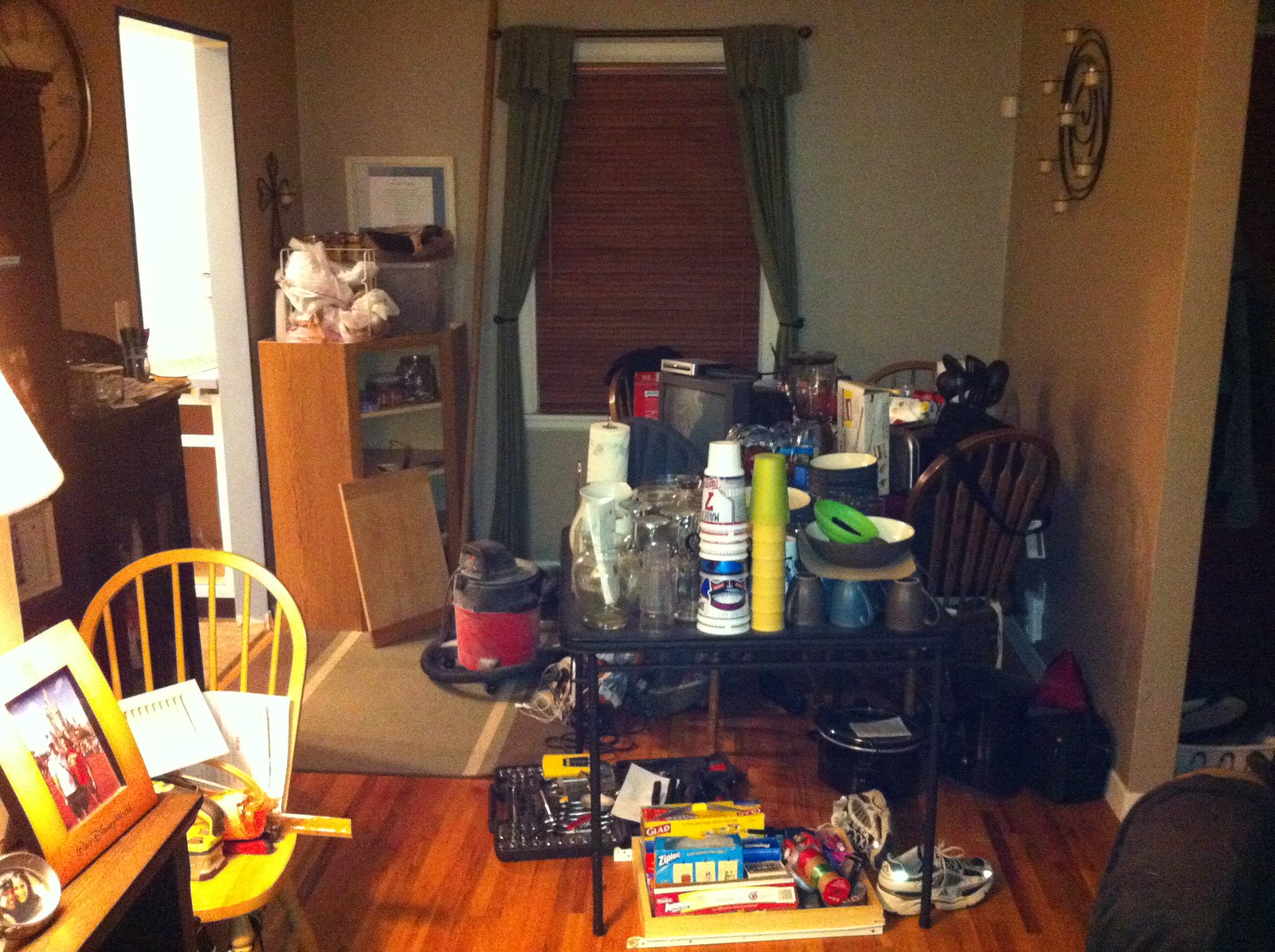The image depicts a cluttered living room filled with various miscellaneous items. 

In the bottom left corner, there is a brown desk adorned with a photo frame, which appears to contain a picture of two people. Also, resting on the desk is a lit lamp emitting a warm yellow glow. Directly behind the desk, a brown colored chair is visible, laden with a variety of items. 

At the center of the image, a black table stands, cluttered with an assortment of objects including multiple cups, plates, bowls, and jars, as well as a napkin dispenser. On this table, an old television and a console box are also visible, adding to the chaos. To the right of this table, more cups and plates can be seen stacked together.

The jars on the table showcase a variety of colors: red, yellow, green, blue, black, and white. To the right of the black table, an artifact is mounted on the wall, surrounded by chairs and positioned near a window. Additional desks are also visible on the left side of the image, contributing further to the room's chaotic atmosphere.